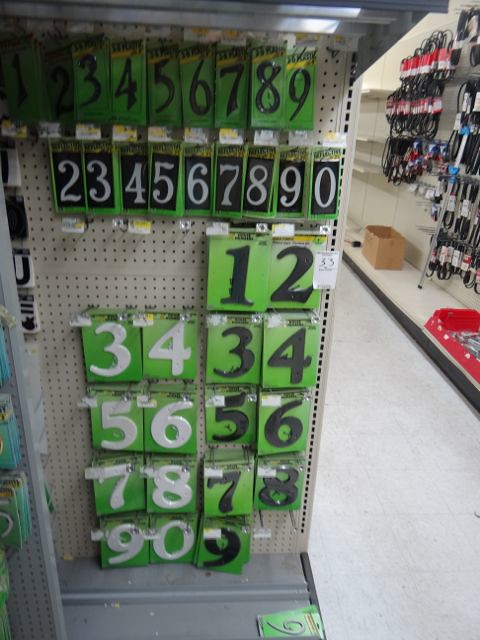This photograph captures an aisle in the hardware section of a store with concrete flooring and display shelves. The main focus is on a white pegboard encased in gray, which prominently displays various styles of house numbers. These numbers, designed for mailboxes or house addresses, are organized into rows based on their color schemes and sizes. The top row features black numbers on green packaging, displaying numbers one through nine. The second row showcases white numbers on black backgrounds, covering numbers two through zero, with the number one missing. The third row contains black numbers on green backgrounds, showing only numbers one and two. Additional rows include white and black numbers on green backgrounds, in various combinations: white numbers three and four, black numbers three and four, white numbers five and six, black numbers five and six, white numbers seven and eight, black numbers seven and eight, white numbers nine and zero, and a black number nine. In the background, there are shelves with black cords and rubber belts of various sizes, likely for appliances or automotive use. Additionally, a cardboard box sits on the bottom shelf to the right, adding a touch of everyday store clutter to the scene.